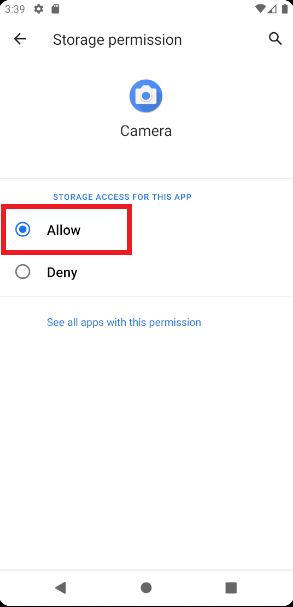The image is a screenshot from a smartphone displaying a permission request interface for an app attempting to access the camera and storage. 

At the very top of the image, the time is shown as 3:39 in the upper left corner. Next to the time, there is a small settings icon shaped like a gear, followed by a folder-shaped icon. To the far right, the signal strength icon, Wi-Fi icon, and battery life indicator are visible.

Just below this top bar, there is a left-pointing arrow labeled "Storage Permission," and to its right, there is a magnifying glass icon indicating search functionality. Below this, a camera icon is present with the label "Camera" beneath it, followed by a thin horizontal border.

The next section features the title "Storage Access for this app" in small blue letters. This section provides two options: "Allow" and "Deny." The "Allow" option is prominently displayed within a red rectangle and is selected with a blue dot.

Below this, there's another horizontal line containing the text "See All Apps with this permission." At the very bottom of the screen are three icons: a left arrow, a small gray dot, and a square, likely representing navigation controls.

**Caption**:
"A smartphone screen displaying a permission request interface for an app seeking access to the camera and storage. Key interface elements include the time displayed as 3:39, icons for settings, folder, signal strength, Wi-Fi, and battery life at the top of the screen. The permission request features clear options to 'Allow' or 'Deny' access, with the 'Allow' option being selected. Navigation controls are located at the bottom of the screen."